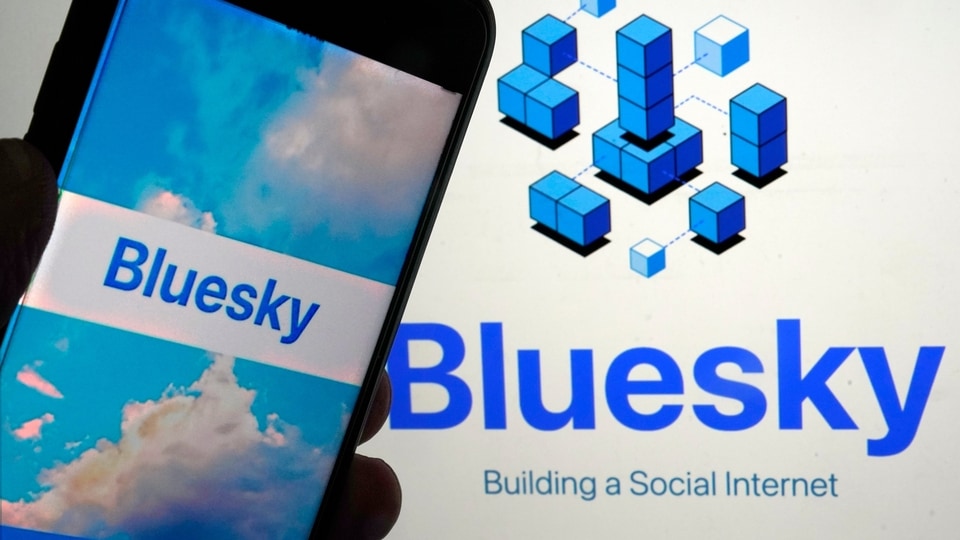The banner for the social media service "Blue Sky" is rectangular with a white background. The top and bottom sides are twice as long as the left and right sides. On the left side, there is a picture of a man holding a black smartphone. The smartphone screen displays a blue sky with clouds and a white banner with blue text that reads "Blue Sky." On the right side of the banner, there is blue text that says "Blue Sky" and below it in smaller font, "Building a Social Internet." The center of the banner features a graphic of multiple blue squares with black borders arranged in various configurations. Some squares are stacked in piles of three, while others form rows of four, and dotted blue lines connect the different shapes, symbolizing the concept of building a social internet.